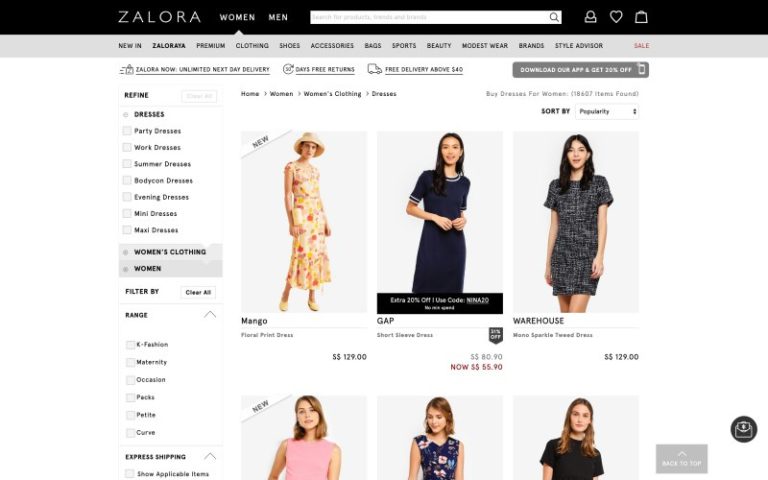This is the web page of a clothing company named Zalora, specializing in both women's and men's apparel. The site prominently displays six images showcasing a variety of garments. Along the left-hand side of the page, there is a detailed but small-printed key categorizing dresses into types such as party dresses, work dresses, summer dresses, bodycon dresses, evening dresses, mini dresses, and maxi dresses. Although the term "bodycon" might be unfamiliar, it typically refers to tightly-fitted dresses designed to accentuate the figure. The dresses vary widely, including options with long sleeves, short sleeves, and very short lengths. The overall impression is that these dresses are targeted at a younger demographic, as evidenced by the youthful appearance of the models wearing them.